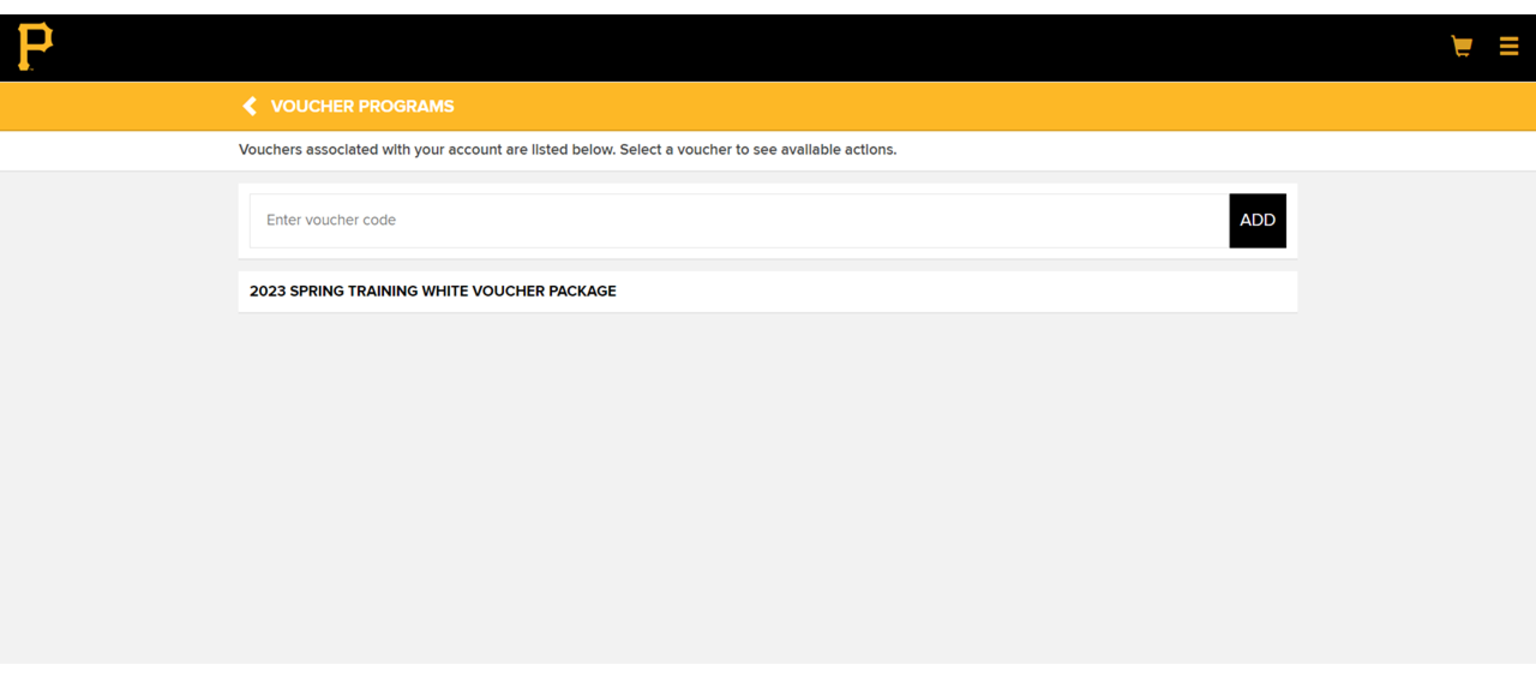The image displays a website layout with a structured, multi-colored header and a centralized search functionality. At the very top of the page, there's a thin blue line running horizontally across. Below this, a one-inch thick black bar spans the full width of the page, containing a yellow "P" icon in the left-hand corner and a yellow shopping cart icon on the right. This cart icon features three horizontal lines stacked atop each other.

Directly below the black bar is a slightly thinner yellow bar, extending across the page. This yellow bar includes a white leftward pointing arrow icon and the text "Voucher Programs" in white, positioned centrally. Beneath the yellow bar, a thinner white bar follows, displaying the text, "Vouchers associated with your account are listed below. Select a voucher to see available options," in black.

The remaining portion of the page is dominated by a large gray box. Centered within this box is a white search bar containing the placeholder text "Enter Voucher Code" in gray. Adjacent to the search bar's right is a black button with "ADO" written in white. Below this, another white bar presents the text "2023 Spring Training White Voucher Package" in black. The rest of the gray box appears empty, providing space for further content or user interaction.